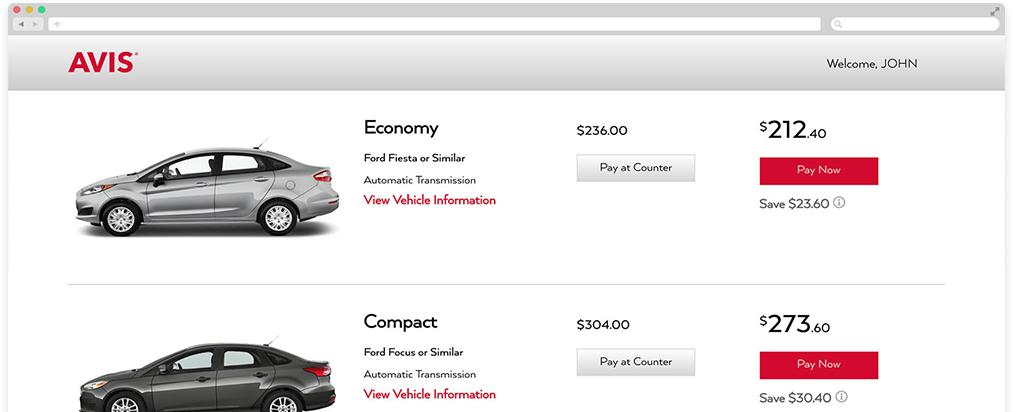On the Avias car rental website, identifiable by its bold red letters at the top, the image showcases a user interface with various navigational elements and car options. The top of the webpage features a dark gray header with familiar browser navigation icons: red, yellow, and green circles in the top left corner, along with arrows for back and forward navigation. To the right of this header is a search bar with a magnifying glass icon, and adjacent to the search bar are screen expansion arrows.

Beneath the header, the main content area displays a sleek gray car, a four-door model with its nose pointing left, categorized under "Economy." The car is identified as a "Ford Fiesta or similar," featuring an automatic transmission. Below the car image, a red link invites users to "View Vehicle Information." Pricing details are prominently displayed: $236.00 under the "Pay at Career" option and $212.40 for the "Pay Now" option.

Further down, there's another car option in the compact category, labeled as a "Ford Focus or similar." This model commands a higher price of $304.00, with a discounted "Pay Now" price of $273.60, accompanied by a distinct red "Pay Now" button.

This detailed interface layout highlights vehicle options available for rental, emphasizing ease of navigation and clear pricing.